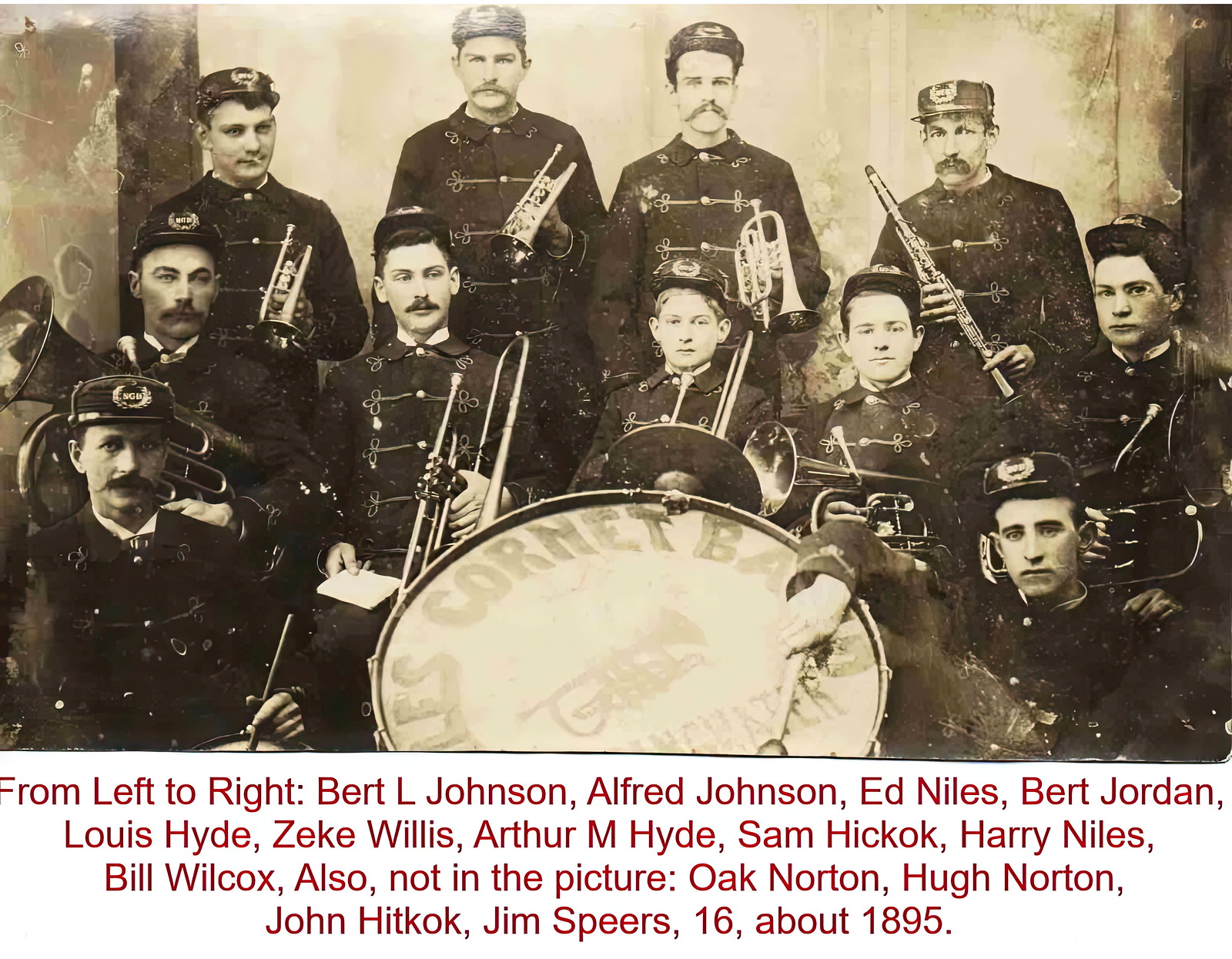This sepia-toned photograph from around 1895 showcases a band composed entirely of men, arranged in three rows. At the front, two individuals are seated with a large drum positioned centrally between them. The middle row contains seated band members, while those in the back row are standing. The men are adorned in dark-colored band uniforms, embellished with gold braiding, and many sport handlebar mustaches.

On the photograph's bottom, a white background with red text lists the names of the band members from left to right: Bert L. Johnson, Alfred Johnson, Ed Niles, Bert Jordan, Louis Hyde, Zeke Willis, Arthur M. Hyde, Sam Hickock, Harry Niles, and Billy Watcox. Notable absentees mentioned include Oak Norton, Hugh Norton, John Hickock, and J.M. Spears. The group appears divided by age; the older men on the left, identifiable by their large beards and mature appearance, contrast with the younger, smoother-faced men on the right. This harmonious yet varied ensemble captures a snapshot of musical camaraderie from the late 19th century.